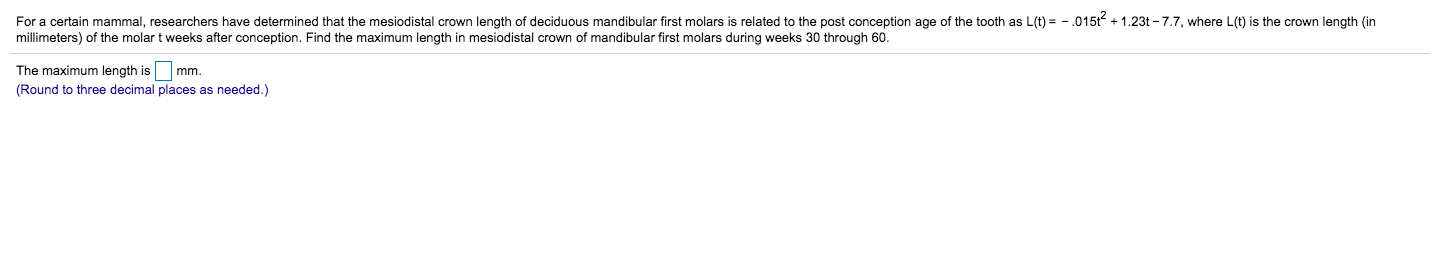Researchers have developed a formula to determine the initial distal crown length of a deciduous mandibular first molar in a specific mammal, relating it to the post-conception age, measured in weeks. The equation \( L(T) = -0.015T^2 + 1.23T - 7.7 \) describes this relationship, where \( L(T) \) represents the crown length in millimeters, and \( T \) is the post-conception age in weeks. To find the maximum crown length of these molars during the gestational period of 30 to 60 weeks, researchers need to apply this quadratic function. The maximum crown length, accurate to two or three decimal places, can then be determined by evaluating the function within the specified timeframe.